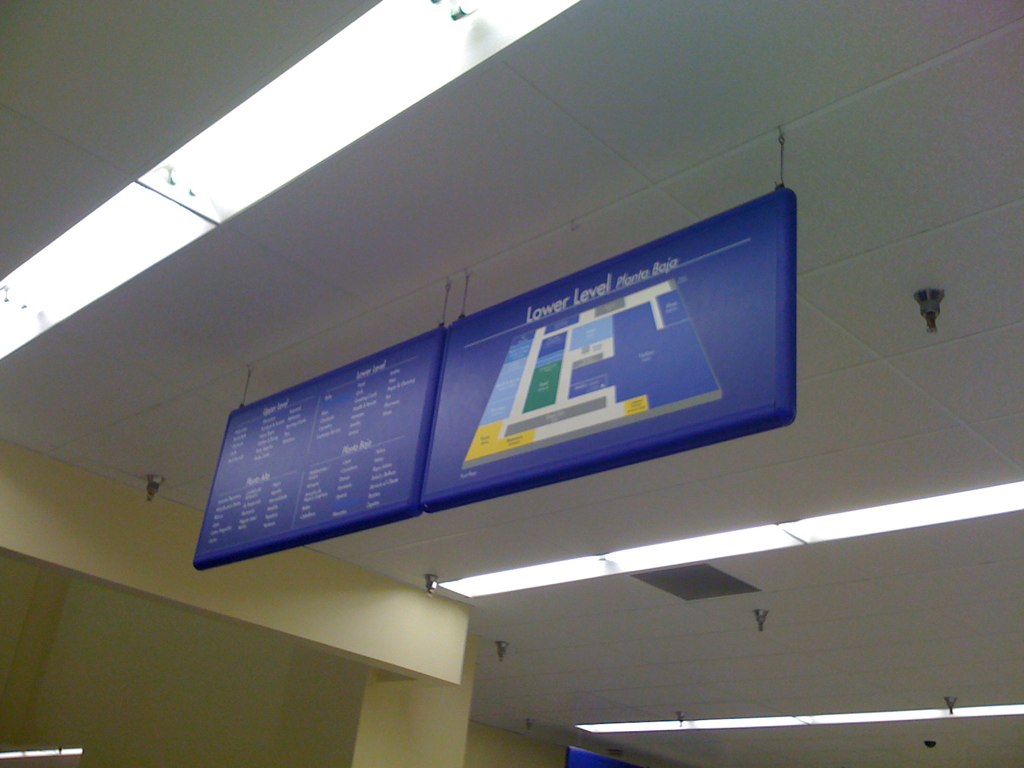This photograph captures the interior of a building, with the camera positioned at a slightly low angle, pointing up towards the ceiling. Hanging prominently from the ceiling are two large blue signs. The sign on the right features a text header that reads "Lower Level" and "Planta Baja," indicating Spanish translation. Below this header, there is a detailed illustration or rendering of the building's layout, serving as a navigational map for visitors to easily locate different rooms and areas within the facility. The leftmost blue sign consists primarily of text, divided into four sections with title headers followed by smaller text, suggesting it is likely a directory listing the names or descriptions of various rooms and buildings. The signs together provide crucial information to help visitors navigate the space efficiently.